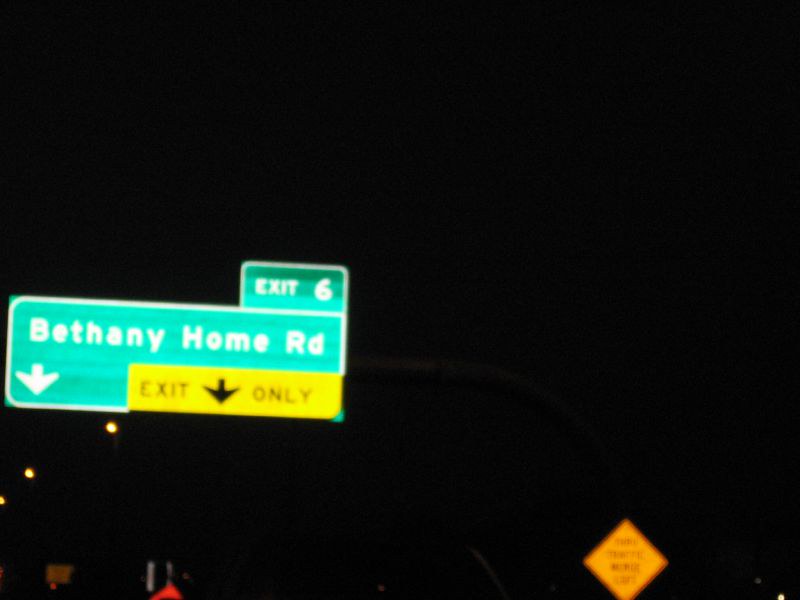The image depicts a nighttime scene on a highway, featuring a prominent green road sign. The large green sign indicates "Exit 6" on a smaller rectangular section at the top, with the words "Bethany Home Road" displayed below it in white letters. A white downward-pointing arrow is situated beneath the text. Adjacent to this is a yellow "Exit Only" sign with a black downward-pointing arrow, indicating lane-specific exit instructions. The sign structure, which supports these signs, has a curving metal pole. Additional elements in the image include two orange diamond-shaped warning signs, one partially visible below the main exit sign and another closer to the right edge of the photo. Due to the darkness and blurriness of the image, the text on these orange signs is unclear, but they likely indicate road work or caution. The dark, pitch-black sky and a couple of visible streetlights underscore the nighttime setting.